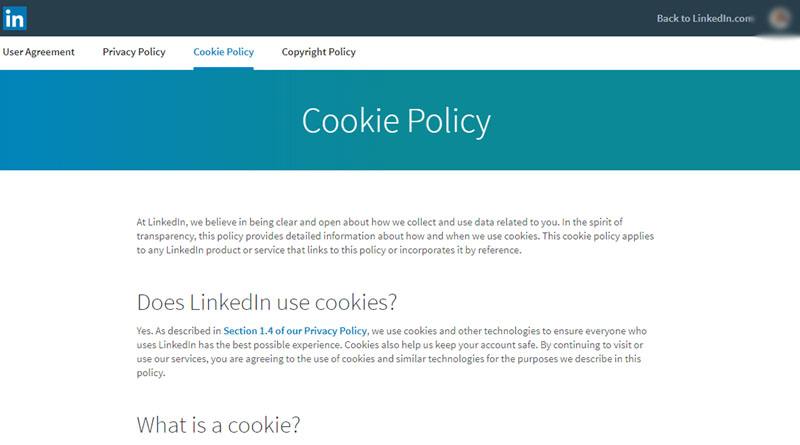This image captures a section of the LinkedIn website specifically focusing on the Cookie Policy page. In the upper left corner, the recognizable LinkedIn logo—a white "in" housed within a blue square—stands out prominently. Opposite this, in the upper right corner, there is a text link labeled "Back to LinkedIn.com" along with a blurred-out profile picture placeholder, indicating the user is logged in but preserving their anonymity. 

Aligned to the left, there is a vertical menu listing several items including "User Agreement," "Privacy Policy," "Cookies Policy," and "Copyright Policy." The "Cookies Policy" is emphasized with a blue underline, signifying that it is the current selection. Below this menu, a horizontally oriented banner features a gradient transitioning from blue on the left to aqua green on the right. Centered in this banner are the words "Cookie Policy," capitalized with a capital "C" and "P."